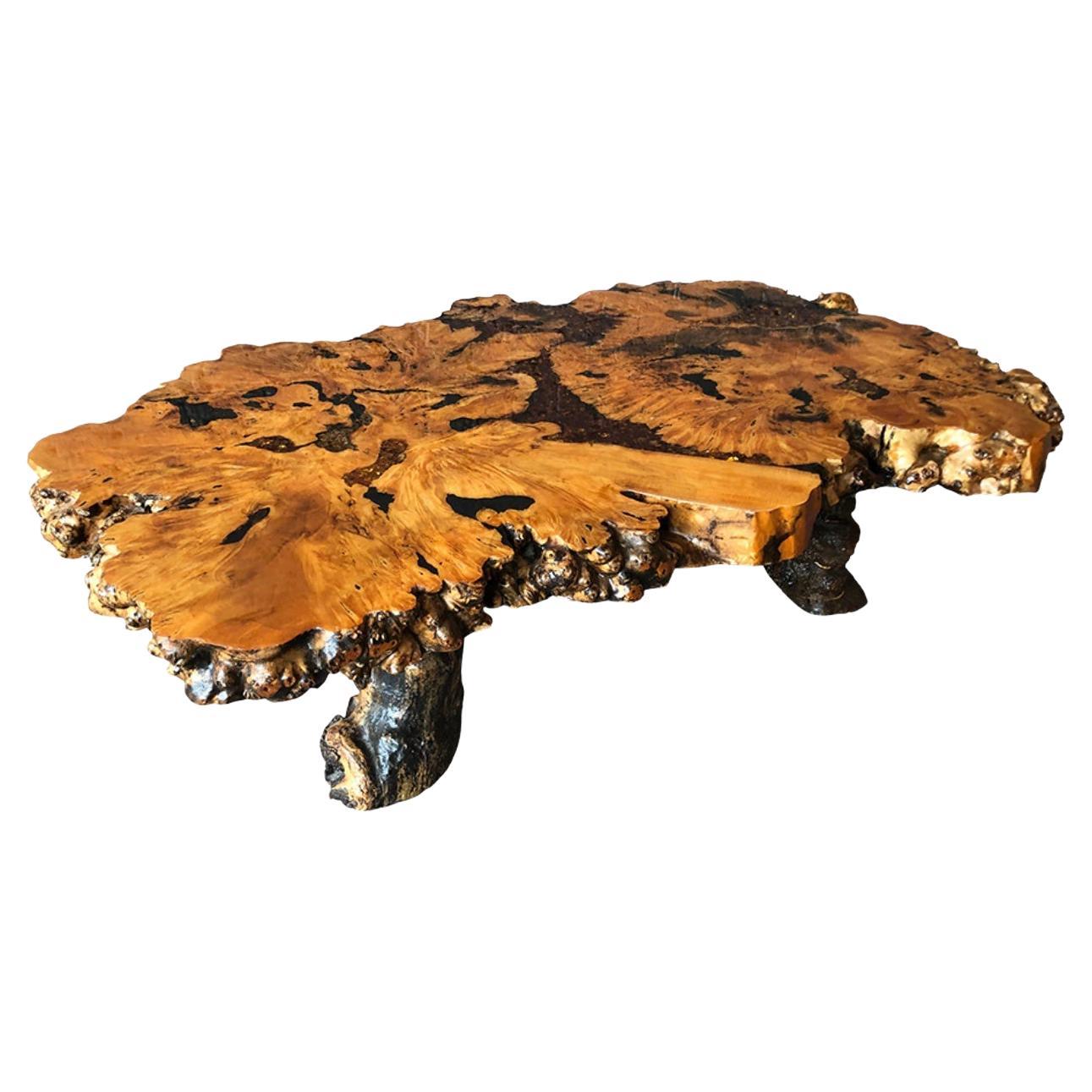This image is a high-detail photograph of a polished wood slice, set against a white background without any defined outline or border. It appears to be a substantial piece of a tree trunk, meticulously sanded, stained, and varnished into a smooth, shiny surface. The finish exudes a warm, darker honey color, showcasing the intricate wood grain and natural markings typical of a tree's inner rings. The piece is quite thick, likely a couple of inches, and seems very hefty. Its distinct wood grain intersperses with black and brown internal structures, possibly resembling a unique, almost ornamental quality. The outer edges retain a rough, black bark-like texture with bulbous contours, contrasting sharply with the polished top. This refined slice, potentially used as a table, rests on brassy legs, giving it a rustic yet sophisticated appearance. The craftsmanship and effort involved in creating such a piece speak to the immense skill and labor required, making this a notable example of woodworking artistry.